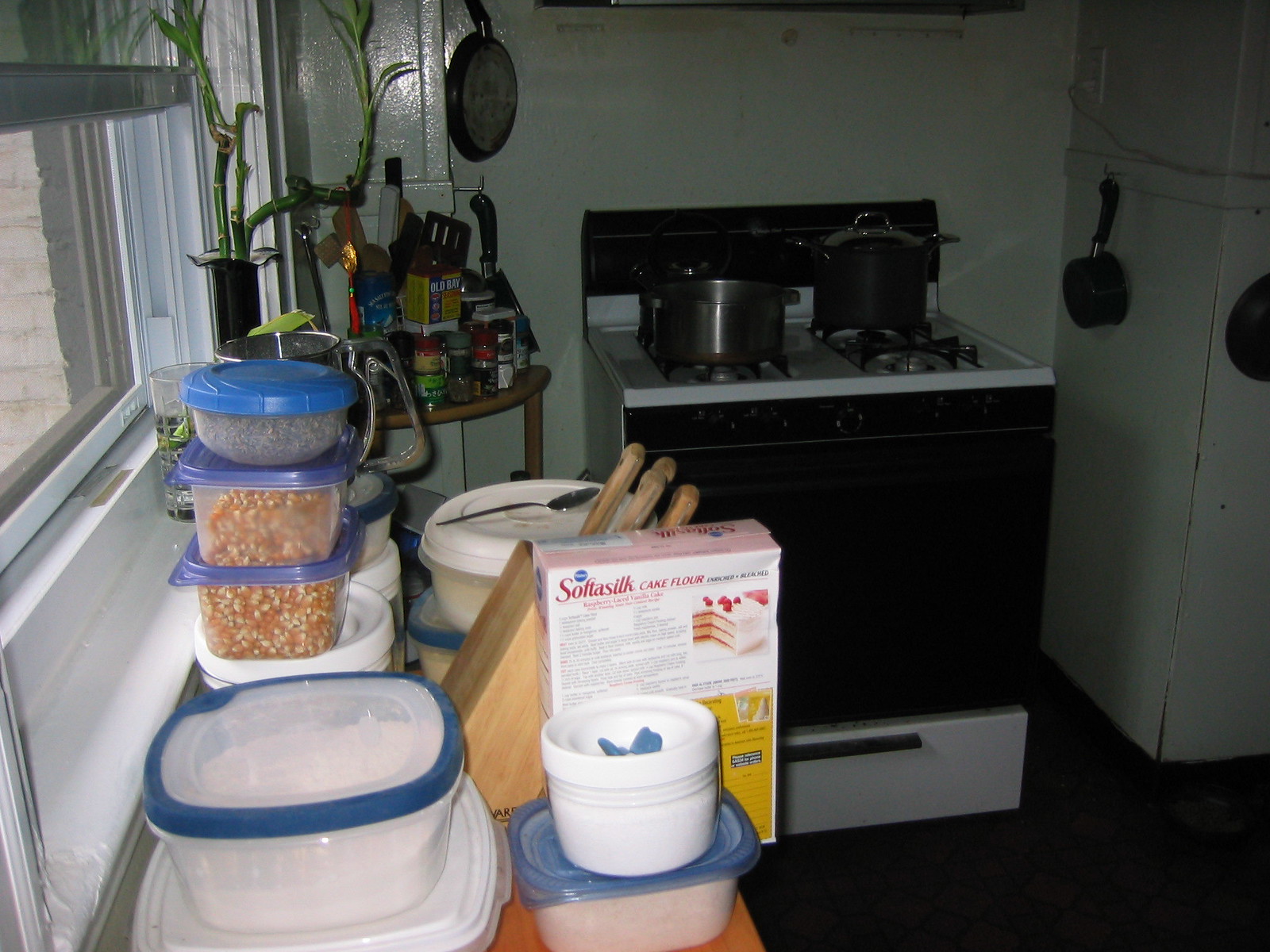This image captures a compact and cluttered kitchen space with limited countertop areas. In the background, a black stove is prominently visible, with two pots resting on its burners. The kitchen layout appears to form an L-shape, as seen from the left side of the photo. On this side, a small countertop is densely packed with various items including Tupperware containers, a box of flour, knives, and other miscellaneous items. The Tupperware containers at the forefront feature blue transparent lids and clear bodies, through which an assortment of red, yellow, and brown cut-up vegetables or possibly cereal is visible. Further in the background, a small plant adds a touch of greenery. Adjacent to the plant, a corner side table is loaded with condiments, spices, and other miscellaneous kitchen essentials, contributing to the busy and congested feel of the space.